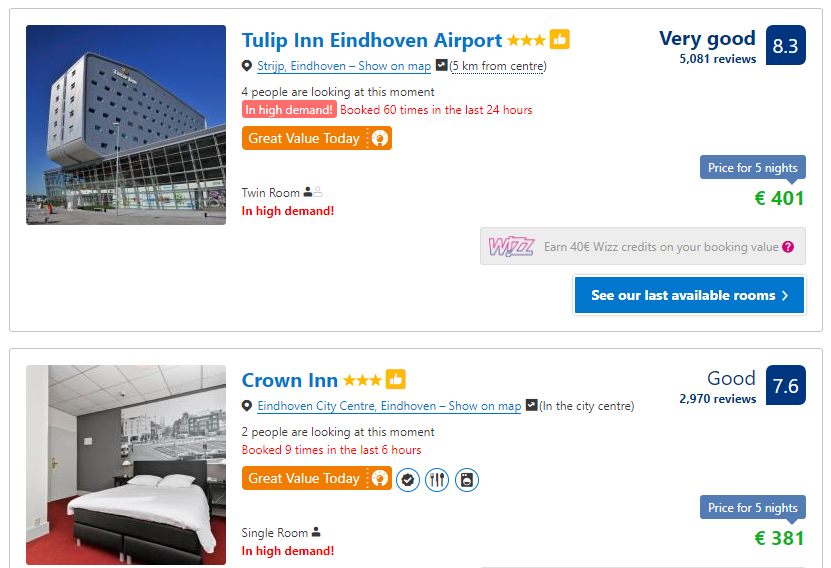In this image, we observe a screenshot from an unspecified hotel booking site displaying several accommodation options. At the top, there is a photo of a distinctive and large hotel, which appears to be uniquely shaped as if balancing atop a building. This hotel is identified as Tulip Inn Eindhoven Airport, situated in Strijp, Eindhoven. According to the details provided, this hotel has received a "Very Good" rating of 8.3 and is noted to be in high demand, having been booked 60 times in the last 24 hours. The website highlights it as a great value option for today, with a twin room available at a price of 401 euros for five nights. A prompt indicates that there are limited rooms left with a message saying, "See our last available rooms."

Below this option, we see another hotel choice featuring a photo of a hotel room with a large bed, red carpeting, and a black and white picture mounted on the wall behind the bed. This hotel is named Crown Inn Eindhoven City Center, located in the city center of Eindhoven. This hotel has a "Good" rating of 7.6 and is currently being viewed by two people. It has been booked nine times in the last six hours. The price for a five-night stay is listed at 381 euros. 

Both listings invite users to explore further details, such as the location on a map and the availability of rooms.